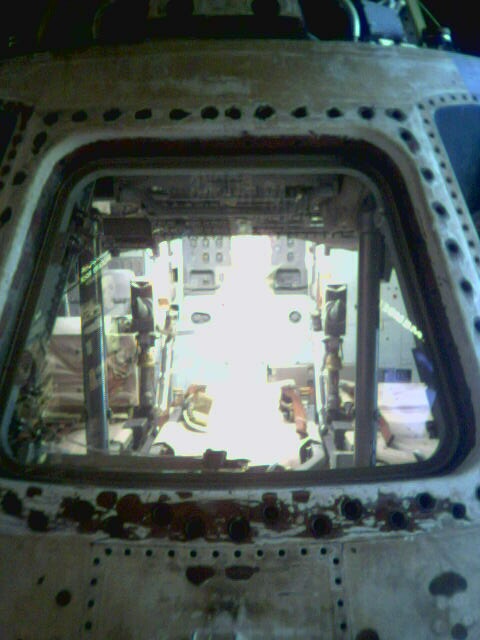This is a close-up photograph capturing the cockpit of an old, possibly military, vehicle or aircraft. The image is taken through a trapezoid-shaped window, framed by a weathered white metal exterior, marked by multiple bolts or rivets. The metal appears rusted and aged, contributing to the vehicle's overall dilapidated look. Inside, the cockpit is filled with various metallic components, including poles, switches, gears, and electronic equipment. The lighting is brighter inside, illuminating the front area equipped with control sticks and multiple panels that might contain gauges, fuses, or buttons. Despite the bright interior, visibility is limited, with darker areas obscuring finer details and allowing only a hint of possible seating arrangements. The right side of the vehicle includes another window, which is opaque and black, preventing any view through it.